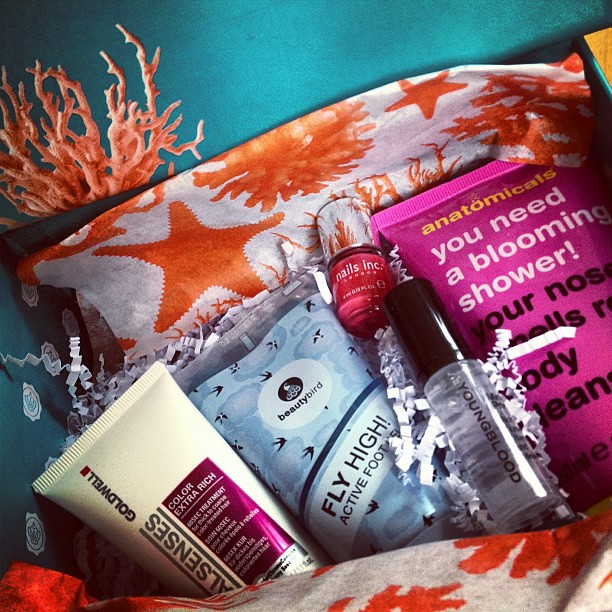The image features a colorful and vibrant arrangement of beauty products and decorative items placed inside a box, reminiscent of a gift basket. Central to the composition are lotion and nail polish bottles, which are arranged around a variety of complementary accessories. The products include a pink tube labeled "Anatomicals You Need a Blooming Shower Your Nose, Body," a transparent bottle with a black cap labeled "Youngblood," a red container with a silver or transparent cover, a blue bottle that reads "Beautybird Fly High Active Foot Gel," and a milky-colored lotion. These items are set against a background with orange and white gift wrap that has star patterns, and flanked by bright orange coral in the top right corner. The entire arrangement is situated on a light blue background that occupies the upper fourth of the image, adding to the bright and inviting feel of the picture. Some confetti and a cloth with fish prints add further texture and interest to the scene, emphasizing a playful and celebratory aesthetic.